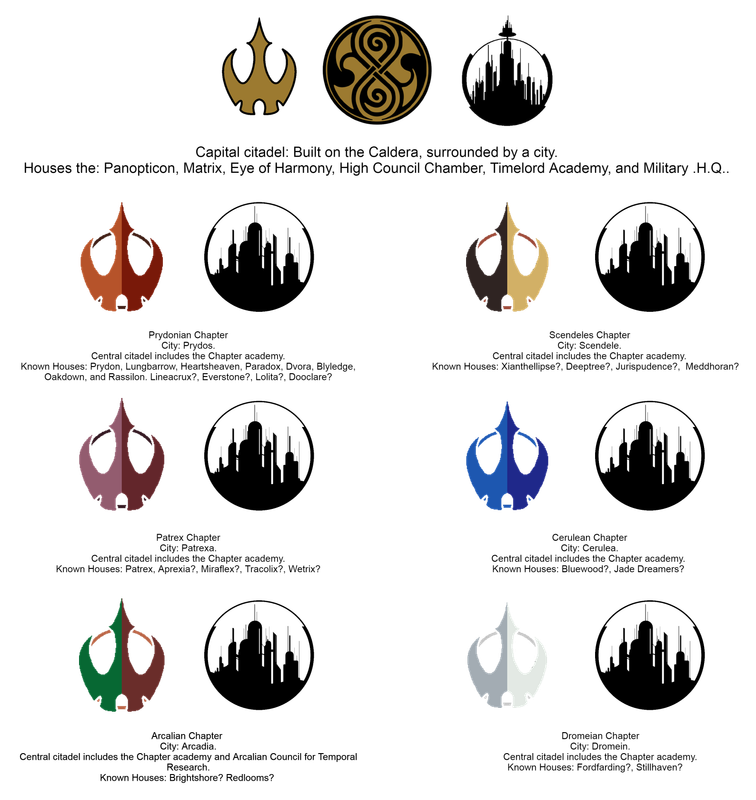The image features an array of various emblems, each accompanied by detailed descriptions. At the top is a trio of distinctive emblems. The leftmost emblem resembles a golden patch with a bird-like design. Next to it is another emblem in gold and black, featuring an intricate design that somewhat resembles the number eight depicted in black. To the right is a circular emblem showcasing a black cityscape. Below this emblem, there's a detailed inscription that reads: "Capitol Citadel built on the caldera surrounded by a city, houses the Panopticon, Matrix, Eye of Harmony, High Council Chamber, Time Lord Academy, and Military Headquarters."

Below this top row are twelve additional emblems, arranged systematically. On the left side, there are three bird-like emblems differentiated by color variations: the top one is orange and red, the middle one is maroon and pink, and the bottom one is green and red. Beside each of these, to their right, are identical black cityscape emblems.

On the right side of the image are three more bird-like emblems. The top emblem is black and gold, followed by one in dual shades of blue, and the bottom one in white and gray. Next to each of these, to their right, are identical black cityscape emblems.

Both rows of emblems are accompanied by further descriptions underneath, providing additional context and details for each symbol.